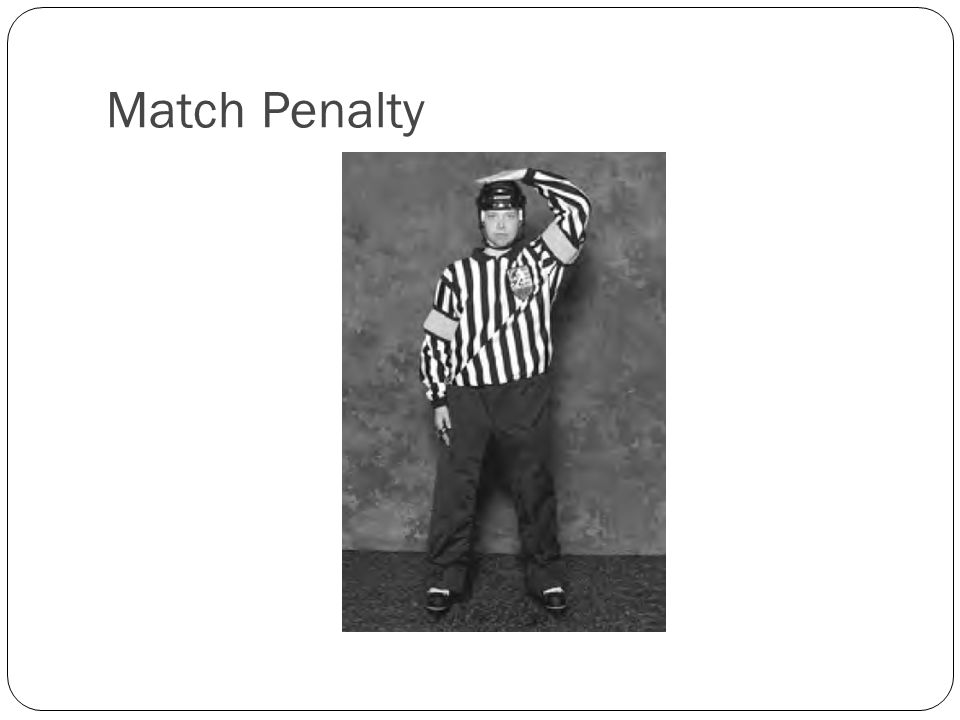This detailed caption combines shared and repeated elements from the snippets provided:

The image is a black and white photograph of a referee, centered on a presentation slide with a thin black border and rounded corners, set against a white background. The referee, identifiable by his classic black and white striped shirt with a patch and armbands, is standing upright, signaling a match penalty. He wears a dark-colored helmet, likely for head protection, and dark pants. The referee has his right hand flat on top of his head and his left hand resting on his hip. The text "match penalty" is displayed in black, horizontal font in the upper left corner of the slide. The overall setting of the photo seems to be indoors, with a wall and floor visible in the background, giving it a stark, minimalist appearance.